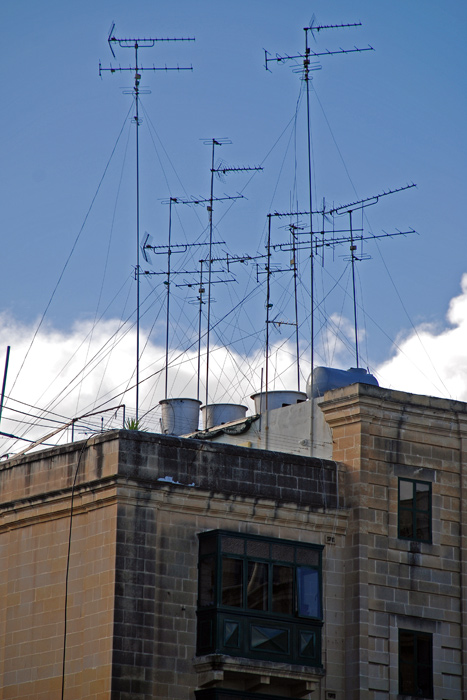The image is a color photograph of two conjoined, weathered brownstone buildings with distinct architectural features. The taller building on the right has a light-colored stone facade, streaked with black algae that highlights its age. It features rows of stone blocks, several prominent windows with dark frames, and a flat roof adorned with various galvanized water tanks. The shorter building on the left steps down about half a story and boasts a distinctive bow window. Crowning both buildings is a chaotic array of at least eight tall antennas with numerous crisscrossing wires, likely for television or communication signals. The roofs also house metal chimneys and a blue tank, possibly for liquid or gas. Against a backdrop of blue sky and white clouds, the buildings present a striking contrast between their worn, neglected surfaces and the high-tech equipment perched at their peaks.